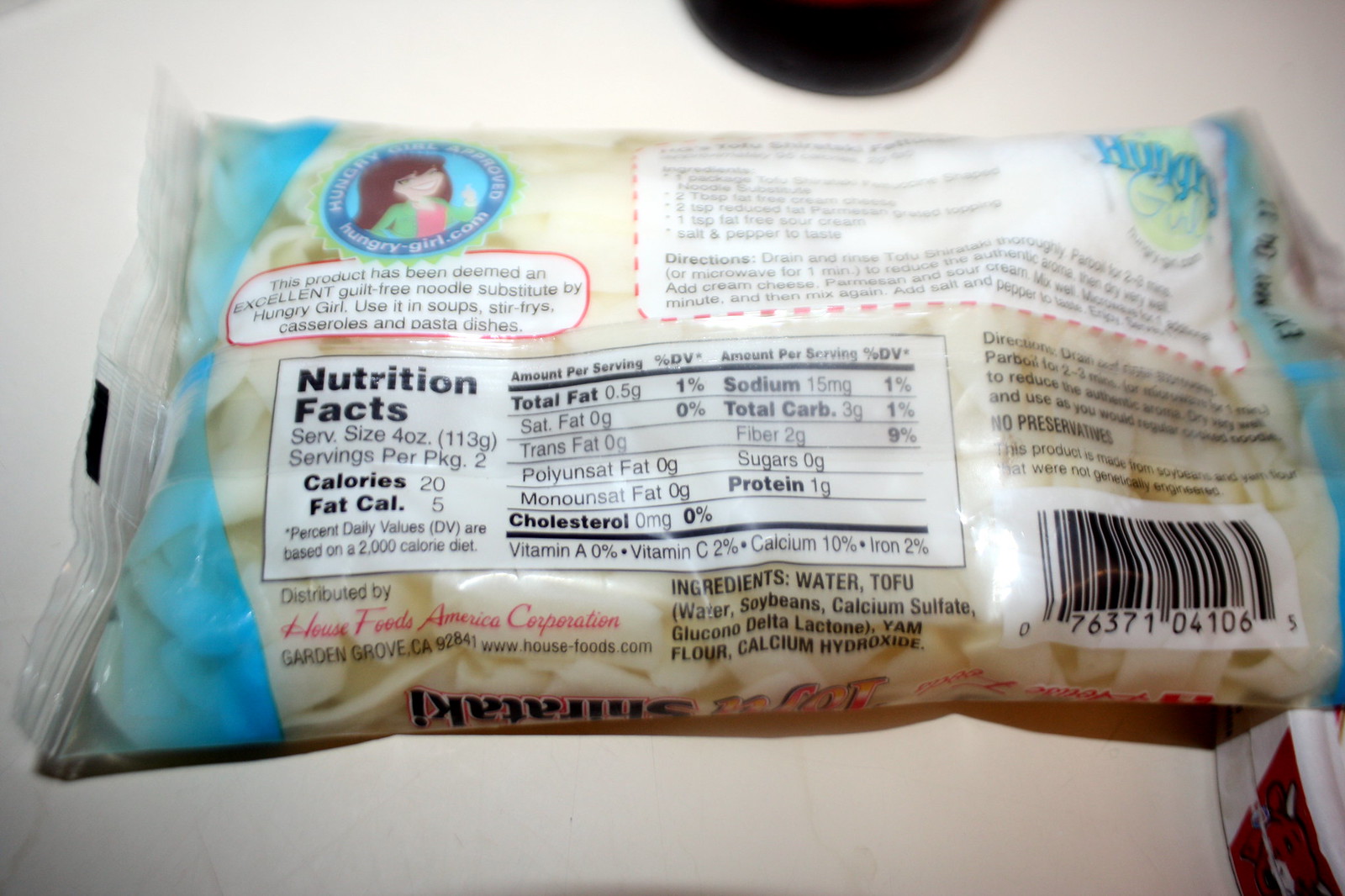A blurry photograph depicts a clear bag with a white product inside, identified as tofu, marketed as an excellent guilt-free noodle substitute by Hungry Girl. The bag features blue accents and a prominent circular logo showcasing a girl with white skin, brown hair, and a green and pink outfit. Detailed nutritional information on a white background with black text is visible, listing serving size as four ounces, with two servings per package. It highlights that the tofu contains 20 calories per serving, 5 of which are from fat, and includes 0.5 grams of total fat, 0 grams of saturated and trans fats, and 0 grams of polyunsaturated fat. Despite the blurriness, a barcode is noticeable. The product is recommended for use in soups, stir-fries, casseroles, and pasta dishes.